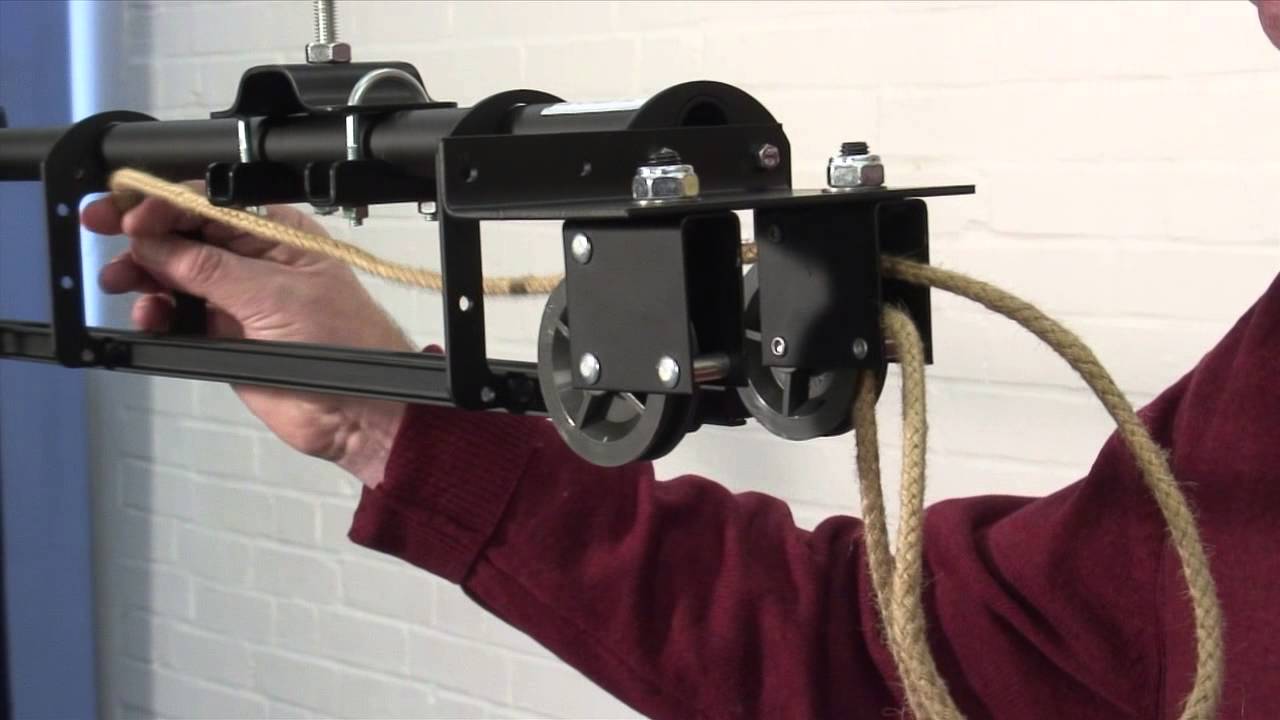In the image, a person's right hand, emerging from the right side, is adjusting a black, intricate pulley system against a backdrop of a white-painted brick wall. The individual, wearing a maroon long-sleeve sweater, guides a yellow rope through the contraption. The machine features multiple poles, levers, and two prominent wheels at its center, one of which is on the right where the rope is being threaded. The entire mechanism is connected by silver bolts and screws, with a cylindrical component partially visible. A faint glimpse of the person's ear or cheek is seen in the upper right corner. The forearm extends across the photograph, emphasizing the active, detailed process of threading the rope through the pulley system. The scene is lit such that there is blue light faintly visible from the left side, suggesting an external light source.